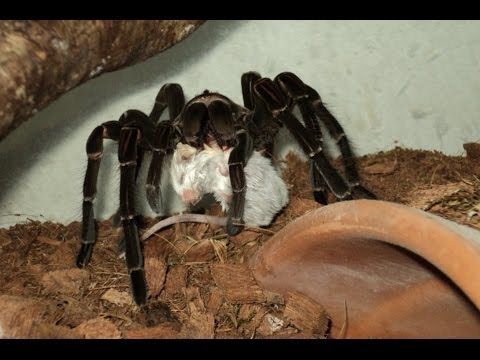The image captures a detailed scene of a large, hairy tarantula standing on medium brown wood chip flooring, inside what seems to be its enclosure. The enclosure features a few decorations, including a dark orange clay pot and wooden branches, with a gray or white wall in the background. The tarantula, recognizable by its black body and distinct white stripes around its leg joints, is depicted in the process of eating a small white mouse, which it holds in its fangs. The mouse, with its grayish pink hairless tail, appears lifeless in the spider's grasp. The photograph highlights the tarantula's fuzzy texture as well as the mouse's fur, giving a vivid portrayal of this moment in the spider's habitat.